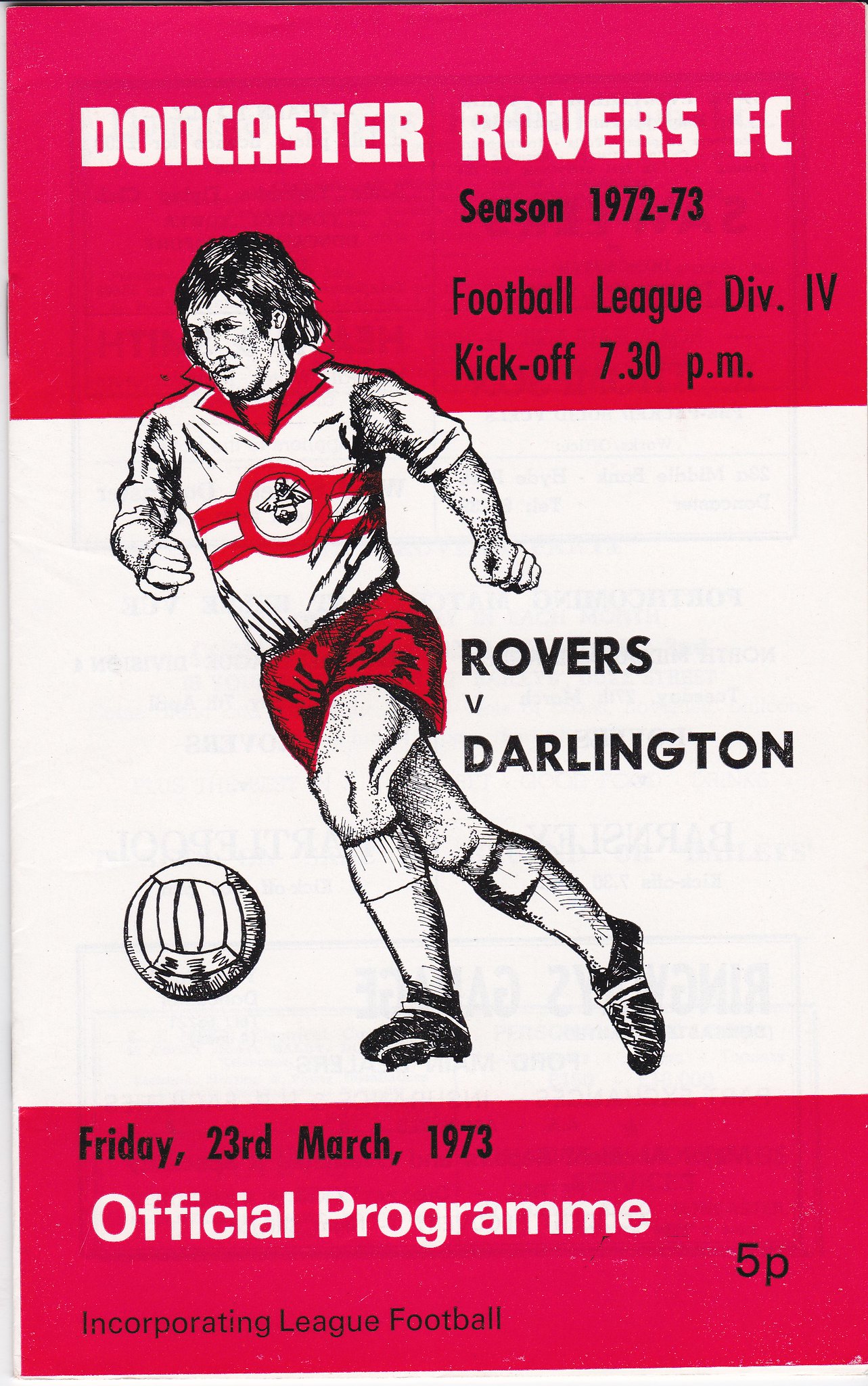The image depicts the cover of an official program from a 1972-73 Football League Division 4 match between Doncaster Rovers FC and Darlington. A central illustration features a soccer player, dressed in a white shirt with a red collar and red shorts, in mid-action with a soccer ball near his left foot. The player's black hair and shading details are evident, and he is set against a white background. Surrounding the illustration, the text is laid out in a structured format. At the top, a bright red rectangular bar with white letters reads "Doncaster Rovers FC." Below, in black font: "Season 1972-73, Football League, Div. IV, Kickoff 7.30 PM." To the right of the player, it states "Rovers vs. Darlington" in black. Another red rectangular banner at the bottom, with black letters, mentions "Friday, 23 March 1973," followed by "Official Program" in white, and "5P" in black. Additional text includes "Incorporating League Football," emphasizing the pamphlet's vintage and official nature.